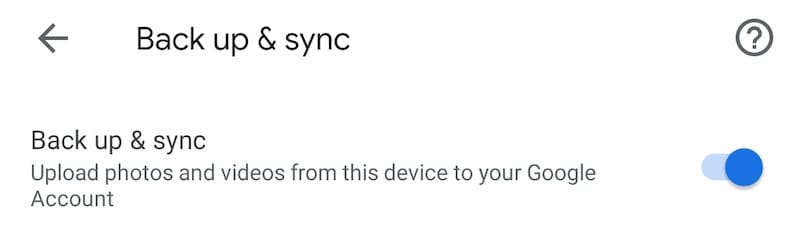A small graphic, likely from a phone or computer, is displayed within a "Backup & Sync" setting. The title "Backup & Sync" (with the ampersand symbol) is prominently shown at the top. To the right of this title is a question mark icon for accessing help, and to the left is a back arrow allowing you to exit the setting. Beneath the title, there's a description that reads: "Upload photos and videos from this device to your Google account." Next to this text, there is a slider button, which is currently toggled to the right, indicated by its blue color. This active setting means that photos and videos from the device will be automatically uploaded to the user's Google account.